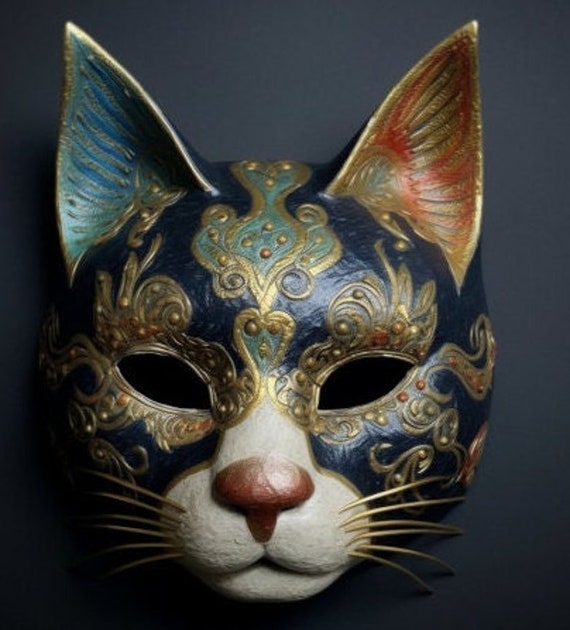This image depicts an intricately designed cat mask. The mask features a delicate blend of colors and textures that create a striking visual impact. The cat's nose is a small, brown protrusion on a white muzzle area, giving it a lifelike touch. Gold-colored whiskers extend from the muzzle, adding a luxurious detail. The eye holes are crafted as black spaces, positioned where the cat's eyes would naturally be.

Both ears of the mask are uniquely colored: the left ear is a deep blue, while the right ear is a vibrant red. Each ear is trimmed with gold and detailed with a golden interior design. The entire mask appears to fit over a cat's face as if the cat itself were donned in an ornamental disguise. The main head section of the mask is a rich blue, adorned with elaborate golden trims and swirling patterns that extend across the top and sides. This ornate and intricately designed piece exudes elegance and artistry.